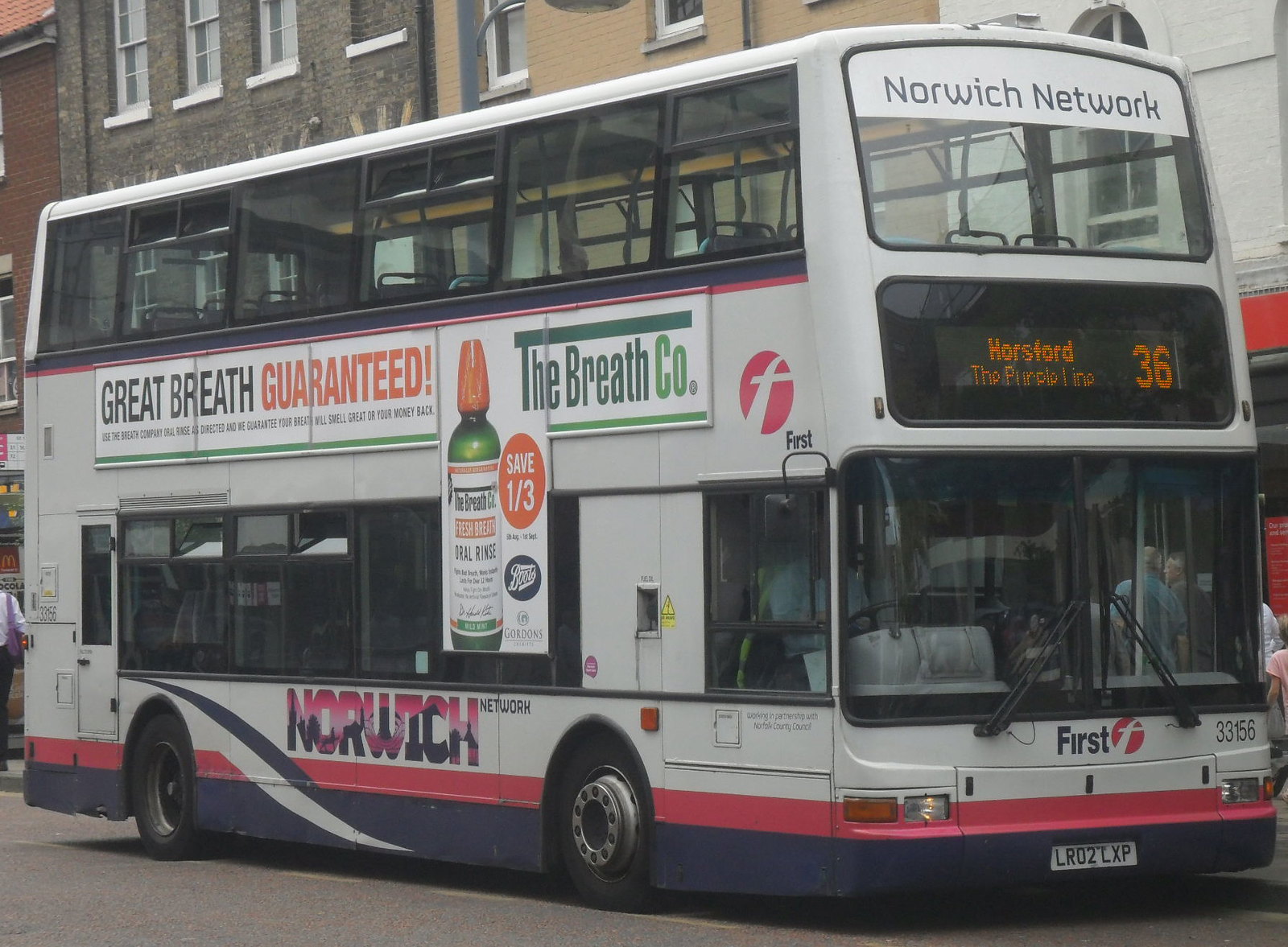The photograph depicts an outdoor scene in the middle of the day, showcasing a parked double-decker bus positioned almost centrally on a solid asphalt surface. The bus, predominantly white with orange and navy blue striping near its base and a pink stripe, prominently displays the text "NORWICH" in large, bold letters, along with "NORWICH NETWORK" on the top deck. The bus's front reads "First" alongside a red circle and white "F," and has a European-style license plate beneath it.

The digital reader board above the driver's window shows "HORSEFORD" and the route number "36" in orange lettering. One side of the bus features an advertisement for The Breath Company with a slogan "Great Breath Guaranteed" and an image of a green bottle of fresh breath oral rinse. Surrounding the bus are a few buildings, and behind it, people walk along the sidewalk. The overall setting appears to be a bus station. The colors in the image range from various shades of gray, blue, pink, red, orange, green, tan, and brown, emphasizing the realistic and detailed nature of the photograph.